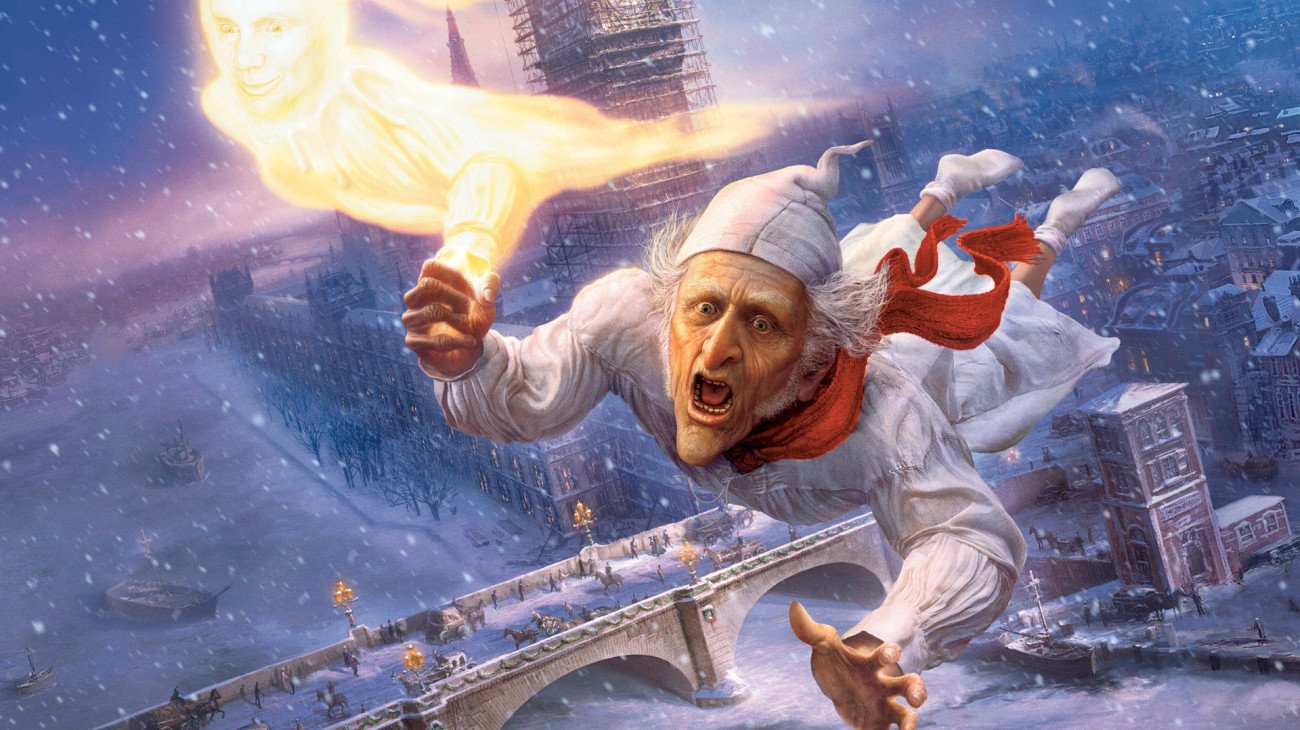This image, likely a still from an animated adaptation of Charles Dickens' "A Christmas Carol," portrays a terrified Mr. Scrooge flying above a snow-covered city. Scrooge, clad in a white nightgown, white socks, a white cap, and a red scarf, clutches the hand of a golden, glowing spirit who appears to be smiling. His mouth is open in a scream, expressing his fear. Below, the cityscape features a bridge bustling with people and horses, a canal with boats, numerous buildings, and another structure adorned with scaffolding. Snowflakes gently fall, adding to the wintry atmosphere of the scene.